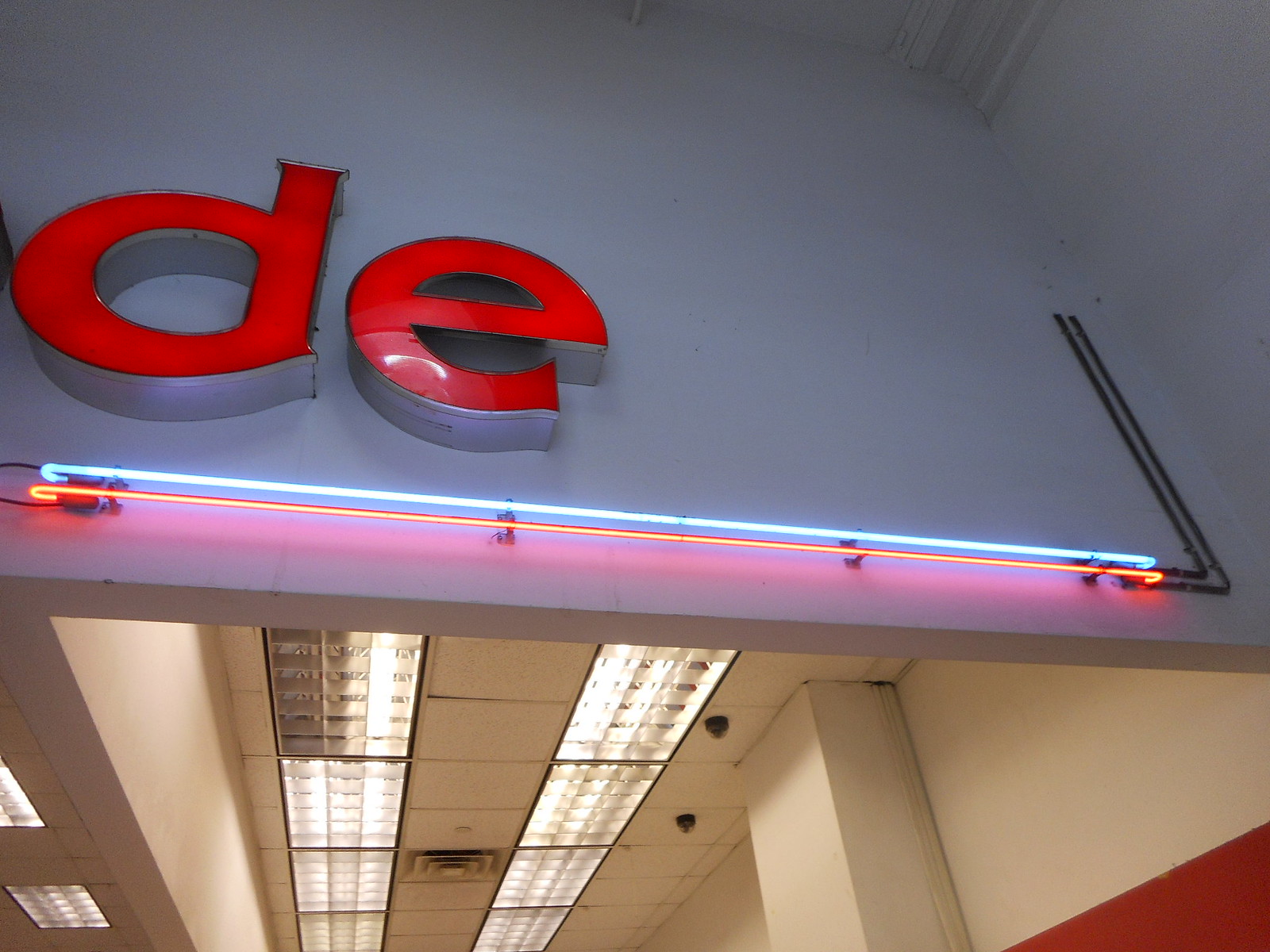In this image, we observe the ceiling of a store-like setting, specifically focusing on the right portion of a wall. The wall displays the bottom segment of a word, revealing only the letters "DE". These letters feature red front faces and gray undersides. The rightmost edge of the wall is adorned with a red stripe, while the remaining wall surface is white. The ceiling above is gray and consists of square tiles, organized neatly into two vertical rows of lights that illuminate the interior. Additionally, the gray wall above the letters includes two distinct lines on the right side; these lines run vertically down before turning left horizontally. The upper line is highlighted with blue light, whereas the lower one is accentuated with orange light.